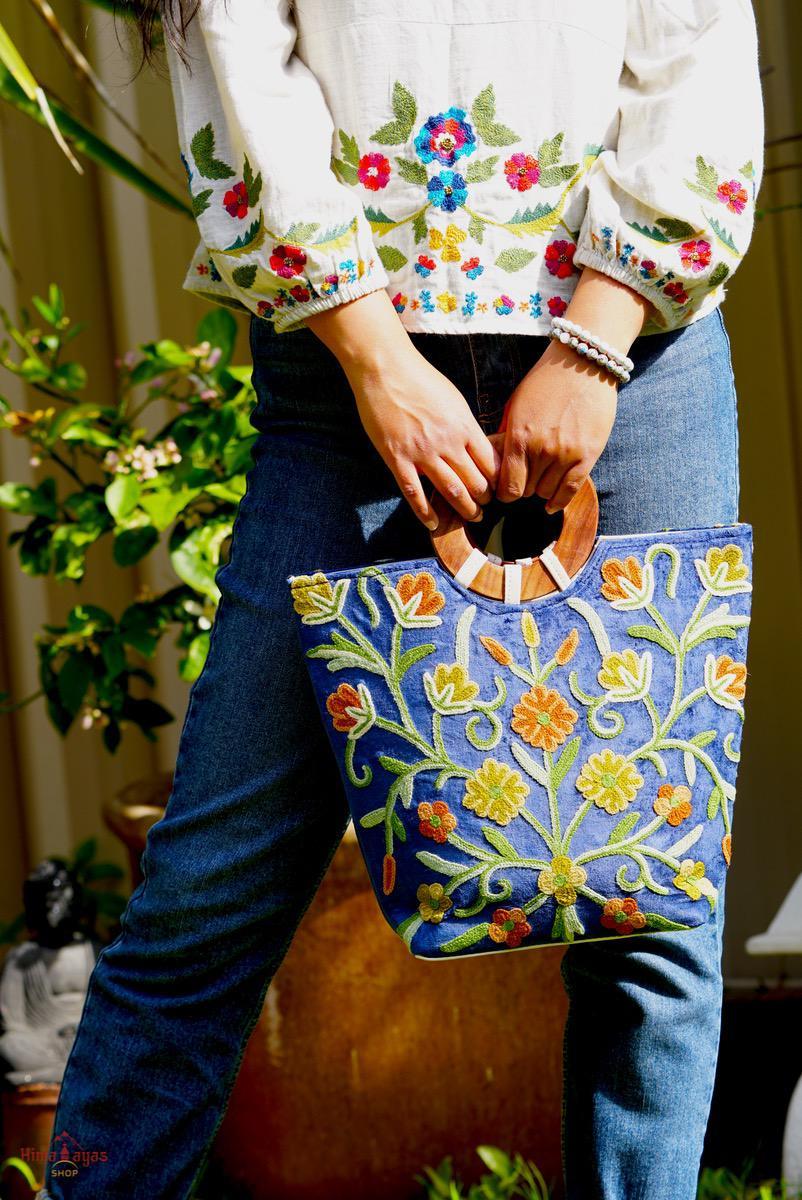This photograph showcases a woman, viewed from her chest to her ankles, holding a beautifully embroidered blue purse behind her back. She stands poised in blue jeans and a white, floral-embroidered blouse that features intricate designs of various colored flowers and greenery, giving a festive, handmade feel. The blouse's floral patterns match the ornate flower designs on the purse, which is accented with green stems, orange petals, and possibly yellow highlights, all swirling in an encompassing, decorative pattern. The purse itself features a distinct round wooden handle for holding. The woman wears a bead bracelet on her left wrist, visible in the shot. In the background, a typical brown ceramic pot with green-leafed plants, some in shadow due to the sun, and a small gray Buddha statue add to the ambiance, making it seem like a garden setting. The composition, likely intended as an advertisement, is visually anchored by the large pot and plant visible between the woman's legs.